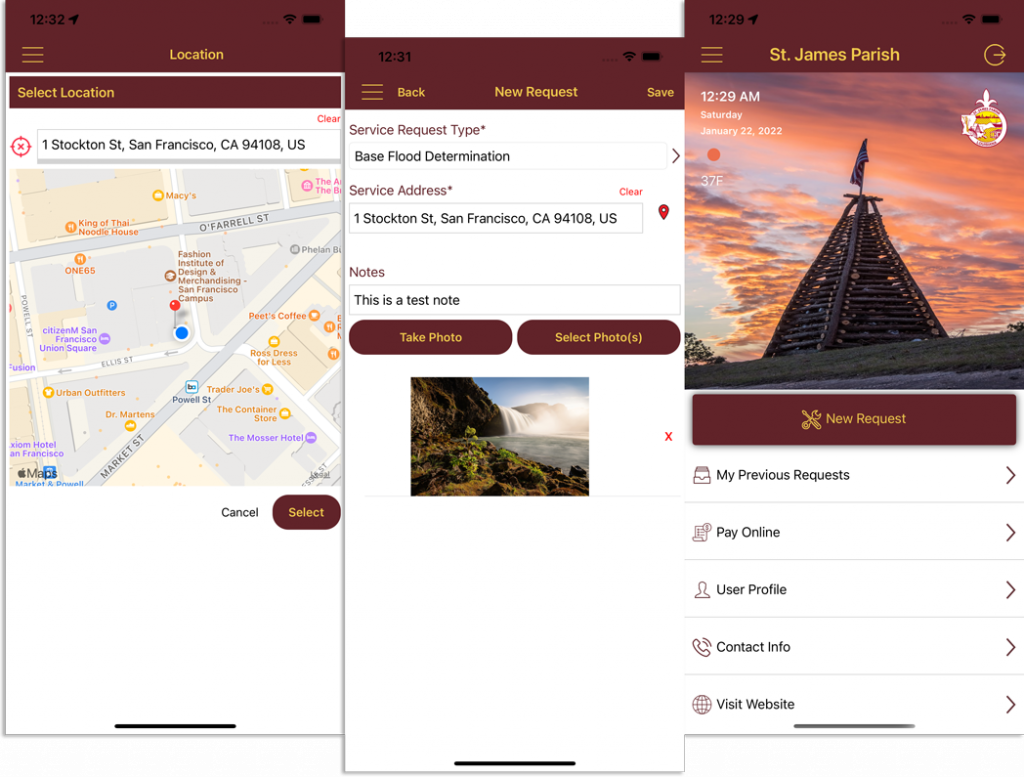Here is an enhanced and detailed caption for the described images:

"Horizontal set of three screenshots detailing an online service request. 

The first screenshot displays the selection of a location through a map interface. The screen reads, 'Select Location,' highlighting '1 Stockton Street, San Francisco, California, 94108, US,' with a corresponding pin on the map. The map is populated with several other labeled locations. Below the map, there are buttons labeled 'Cancel' and 'Select.'

The second screenshot pertains to initiating a new service request. The screen is titled 'New Request' and specifies the 'Service Request Type' as 'Base Flood Determination.' The 'Service Address' is listed as '1 Stockton Street, San Francisco, California, 94108, US.' There is a section for 'Notes' containing the text, 'This is a test note.' Below, options to 'Take Photo' or 'Select Photos' are visible, with an attached photograph of a waterfall.

The third screenshot features 'St. James Parish,' displaying an image of a pyramid-shaped structure constructed from logs, topped with an American flag. The sky behind the structure exhibits a mix of gray and pink clouds during either sunset or sunrise. The timestamp reads '12:29 AM, Saturday, January 22nd, 2022,' with a temperature of '37°F.' Elements at the bottom of the screen include options for 'New Request,' 'My Previous Requests,' 'Pay Online,' 'User Profile,' 'Contact Info,' and 'Visit Website.'"